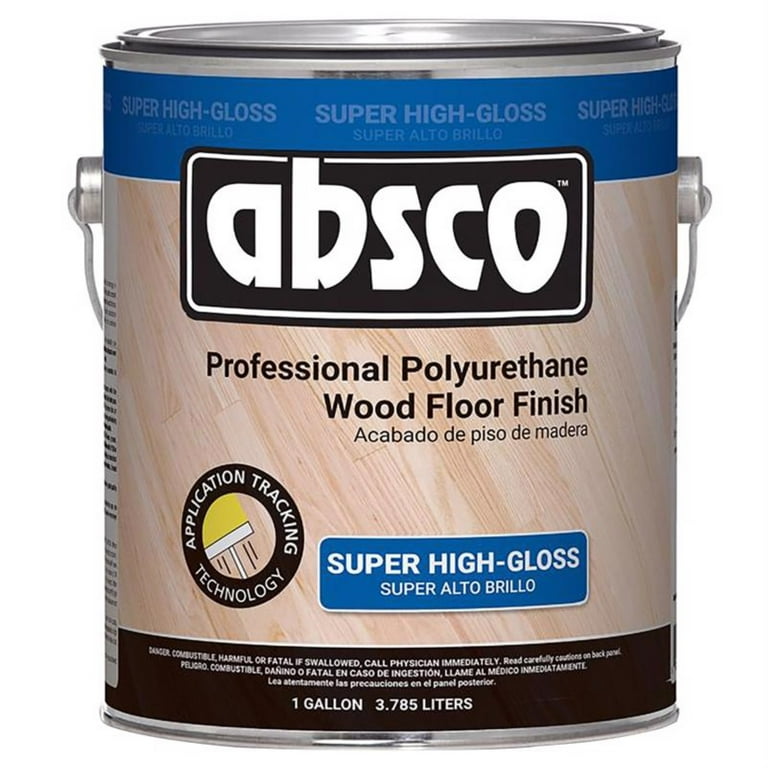This photograph showcases a metal can of wood floor finish produced by ABSCO™. The can has a metal lid and a handle, parts of which are visible behind it. A prominent blue banner at the top reads "Super High Gloss" and "Super Alto Brillo" in Spanish, which is reiterated at the bottom of the can in a rounded rectangle. The product label prominently features the text "Professional Polyurethane Wood Floor Finish" and its Spanish counterpart, "Acabado de Piso de Madera," over a background image of a light wood floor that wraps around the can. To the left of the text, a black circle illustrates "Application Tracking Technology" with an image of a brush applying a yellow finish to the wood. A black banner at the bottom provides volume details, stating "one gallon (3.785 liters)," and includes a safety warning in both English and Spanish: "Danger, combustible, harmful, or fatal if swallowed. Call physician immediately. Read carefully cautions on back panel" and "Peligro, combustible, dañino, o fatal en caso de ingestión. Llame al médico inmediatamente. Lea atentamente las precauciones en el panel posterior." The can’s design is predominantly light and dark brown with blue accents, reflecting its content and branding elements.